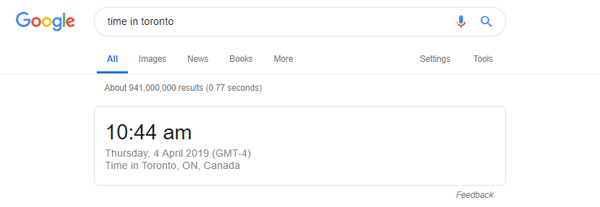Screenshot of an Old-Style Google Search Interface

In this image, we see a screenshot of the Google search interface from April 4, 2019. The recognizable Google logo, featuring its standard primary colors (blue, red, yellow, and green), is prominently displayed on the top left corner. Adjacent to the logo lies the search bar, flanked on its right by a small microphone icon and an hourglass icon, symbolizing voice search and search history, respectively.

Directly beneath the search bar is a horizontal menu showing categories of search results. The “All” category is highlighted in blue and underlined, indicating it as the current selection. Other categories listed include Images, News, Books, More, Settings, and Tools.

The search results section indicates "about 941 million results" found in "0.77 seconds," demonstrating the speed and vast scope of Google's search capabilities. 

Below this, set within a box, the time is stated as "10:44 AM, Thursday, 4 April 2019, GMT-4," with a specific note of the time zone being in Toronto, Ontario County, Canada. There is an option for user feedback at the bottom right corner of this box, labeled "Feedback Set." The remainder of the screen is blank and black, with no visible search result entries.

This image captures an older version of the Google search interface, slightly different from more modern iterations in its layout and design elements.